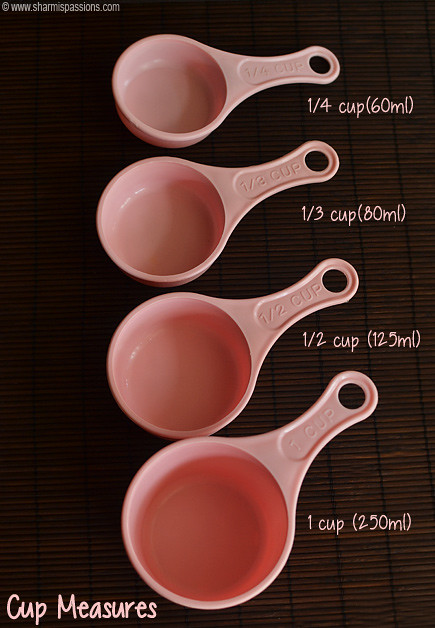This photograph features a set of four beige measuring cups arranged flat on a dark brown surface with a pattern of small lines. At the top of the image, there is the text "www.shamspassions.com." Each measuring cup, viewed from above, has a handle with a circular hole for connecting the set together. The measurements are clearly marked on both the cups and handles in both cups and milliliters: the largest cup at the bottom indicates "1 cup" (250 milliliters), followed by "1/2 cup" (125 milliliters), "1/3 cup" (80 milliliters), and "1/4 cup" (60 milliliters) as you move upwards. At the very bottom left of the photograph, it reads "cup measures."